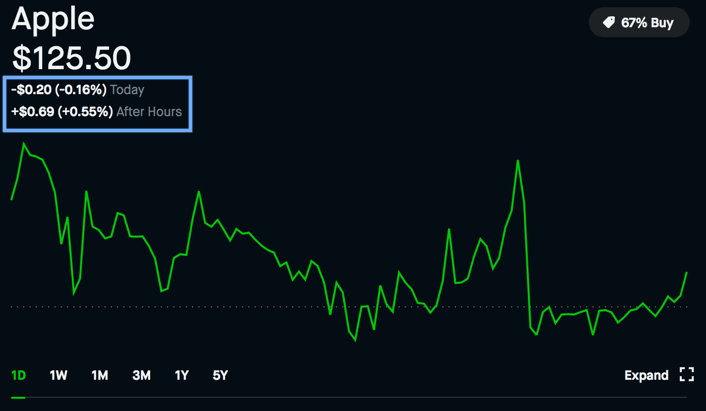The image displays a dark-themed financial statistics page focused on Apple's stock performance. In the upper left corner, the word "Apple" is prominently displayed in large white text, followed by a dollar sign and "125.50" indicating the stock's price. Below this, a blue-bordered box shows a decrease of "0.20" and "0.16%" in white text, with "today" mentioned underneath. Further down, it indicates an "after hours" increase of "0.69" and "0.55%" in the same format.

The main feature of the image is a green line chart depicting the fluctuating stock price trends. In the upper right corner, the text "67% buy" is displayed in white alongside a small grayish button. Toward the bottom left, a green "1D" signifies a one-day view of the data, with additional time frame options "1W, 1M, 3M, 1Y, 5Y" listed. On the right, the word "expand" appears with an icon of four corners forming a square, suggesting an option to enlarge the chart.